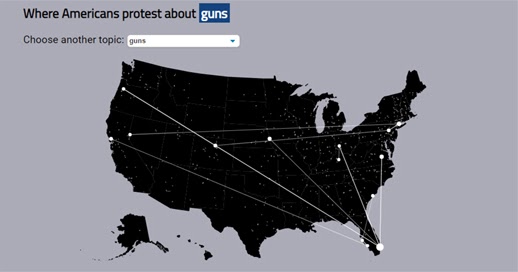A detailed map graphic displays the continental United States in black against a gray background, with smaller inset illustrations of Alaska and Hawaii positioned below where Mexico would typically be. These insets are situated beneath Arizona and New Mexico. The graphic is titled "Where Americans Protest About Guns," and includes a dropdown menu with "guns" selected, implying other protest topics can be chosen.

Marked on the map are specific locations where protests against guns occur, including notable cities such as Portland, Oregon; San Francisco, California; Chicago, Illinois; and several cities in Florida. Dots also appear in Washington state and in the central United States, potentially indicating cities like Denver, Colorado, and St. Louis, Missouri. The visual suggests that while gun protests are concentrated in common metropolitan areas, a few also take place within the central regions of the country.